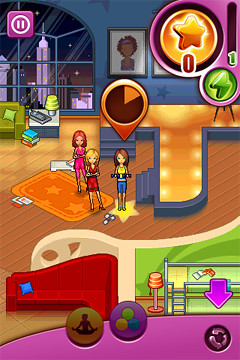This detailed screenshot from a colorful mobile game or web browser flash game, likely set in a New York loft apartment, features a distinctly cartoonish 2D art style. At the center of the room, three female characters face the viewer: the one in the middle is a blonde woman wearing a small red dress and red high heels, with her arms folded. To her left (though slightly behind) stands a woman with red hair, sporting a pink jumpsuit and also folding her arms. On the right stands a brunette in a yellow tank top and small blue shorts. These characters are positioned near a lit-up fashion runway amidst sparse furnishings, including a large window revealing the Empire State Building against a starry night sky. The room has wooden flooring, bright orange carpeting, and bunk beds visible in another section. The game interface features various UI elements: a purple square with a pause icon in the upper left corner, a star meter and a green lightning bolt icon in the upper right, and two circular buttons (one depicting a yoga pose and another with three circles in a triangle) in the lower right corner. Additional interface buttons, including a pink arrow and a recycle button, adorn the edges, further indicating a dynamic simulation game environment.